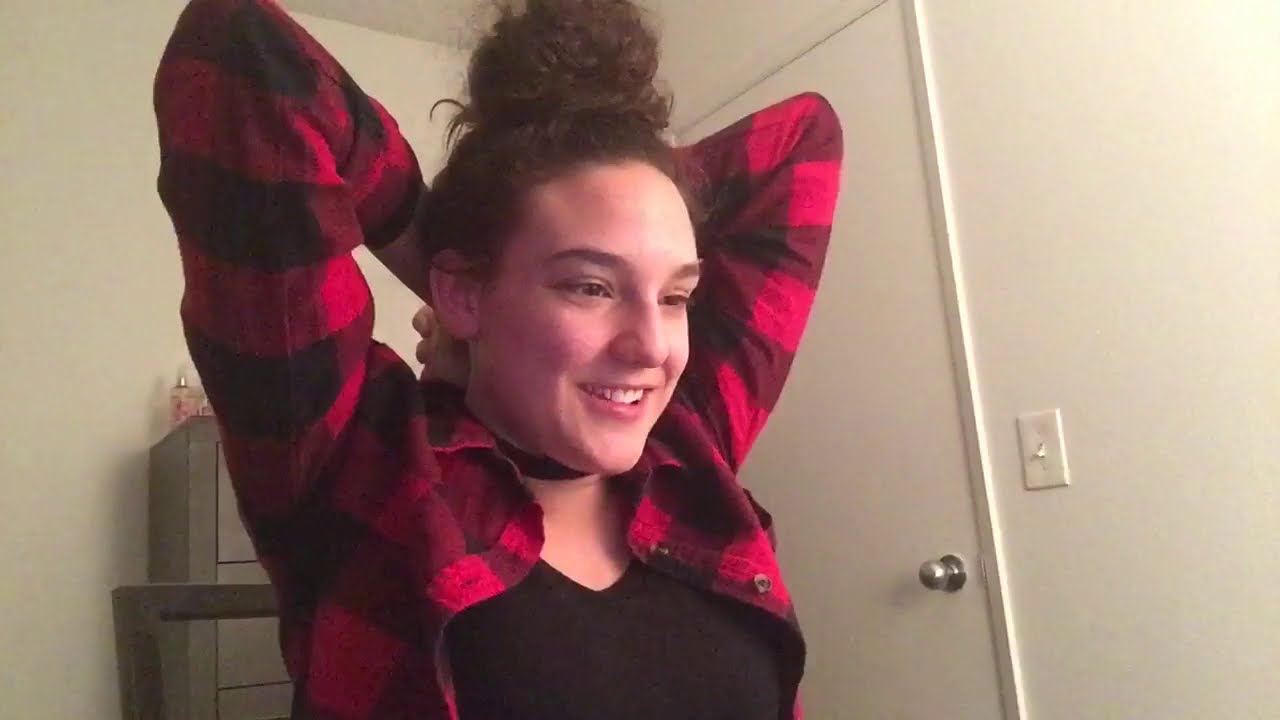In the image, a young woman, appearing to be around 20 years old, stands centrally in what seems to be an indoor setting, likely a bedroom. Captured from the chest up, she faces forward and slightly to the right, with her dark brown hair tied up in a bun on top of her head. She wears a red and black plaid long-sleeve shirt over a black V-neck t-shirt. A black band is visible around her neck. She stands with both arms raised behind her head, hands resting on the back of her neck, and her elbows pointed upwards. She has a half-smile, with her mouth slightly open, showing her upper teeth, and she gazes slightly downward to the right.

Behind her, to the left, is a gray dresser with perfume bottles on top, and to her right is a white or cream-colored wall with a light switch and a door with a silver knob. The overall color palette of the image includes shades of white, gray, pink, red, black, tan, and silver. The photograph, likely taken as a selfie, exudes a casual and relaxed vibe, suitable for social media sharing.